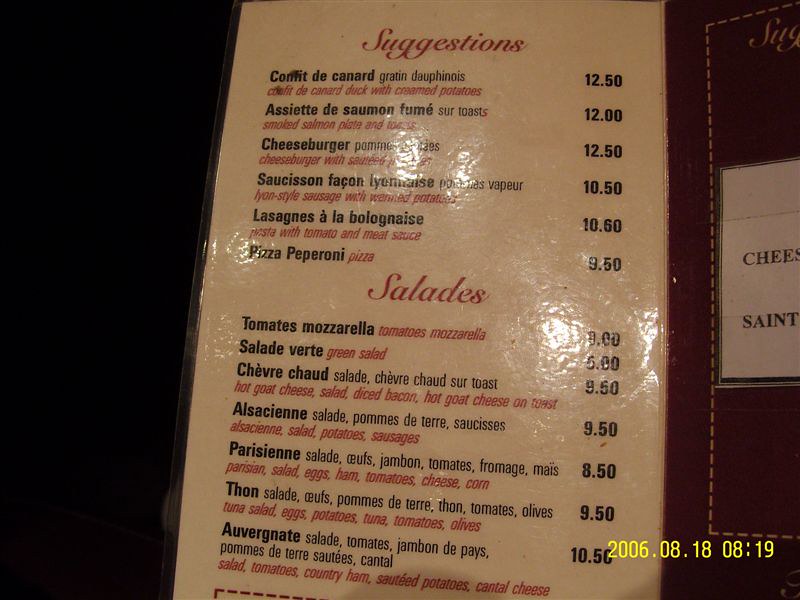The image depicts a restaurant menu presented in a luxurious holder crafted to resemble leather or faux leather. The menu is placed on the left side within this elegant folder, protected by a plastic cover. To the right within the folder, partial text can be seen, beginning with 'CH-E-E-S' and followed by 'Saint,' although the significance of this text remains unclear.

The menu itself is dated August 18, 2006, with a timestamp of 8:19, though it's ambiguous whether this refers to AM or PM. The contents of the menu are primarily in English, though it features certain dish names in another language, which appears to be Italian. Menu options include classics such as lasagna, cheeseburgers, and pizza. Given these items, it can be inferred that the restaurant likely specializes in Italian cuisine.

A notable observation is that the menu prices are reflective of the time, significantly lower than contemporary prices due to inflation, as evidenced by a pizza priced at just $9.50. This menu provides not only a glimpse into the restaurant's offerings but also serves as a historical artifact from 2006.